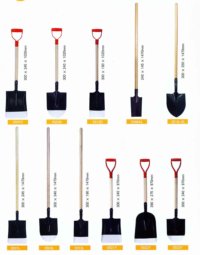The image displays a collection of 11 distinct spades arranged in two rows against a plain white background. The top row consists of five spades and the bottom row features six spades. Each spade has a black blade and a long wooden handle, though the handle lengths vary. Notably, the first three spades in the top row and the last three spades in the bottom row have red handles, while the remaining spades consist solely of a long wooden pole without any handles. The spades display an assortment of blade shapes, including square scoop shovels, thin rectangular shovels, and pointed shovels. Labels are positioned beside each spade, and there is a yellow label beneath each spade, though the text is too small to be read.